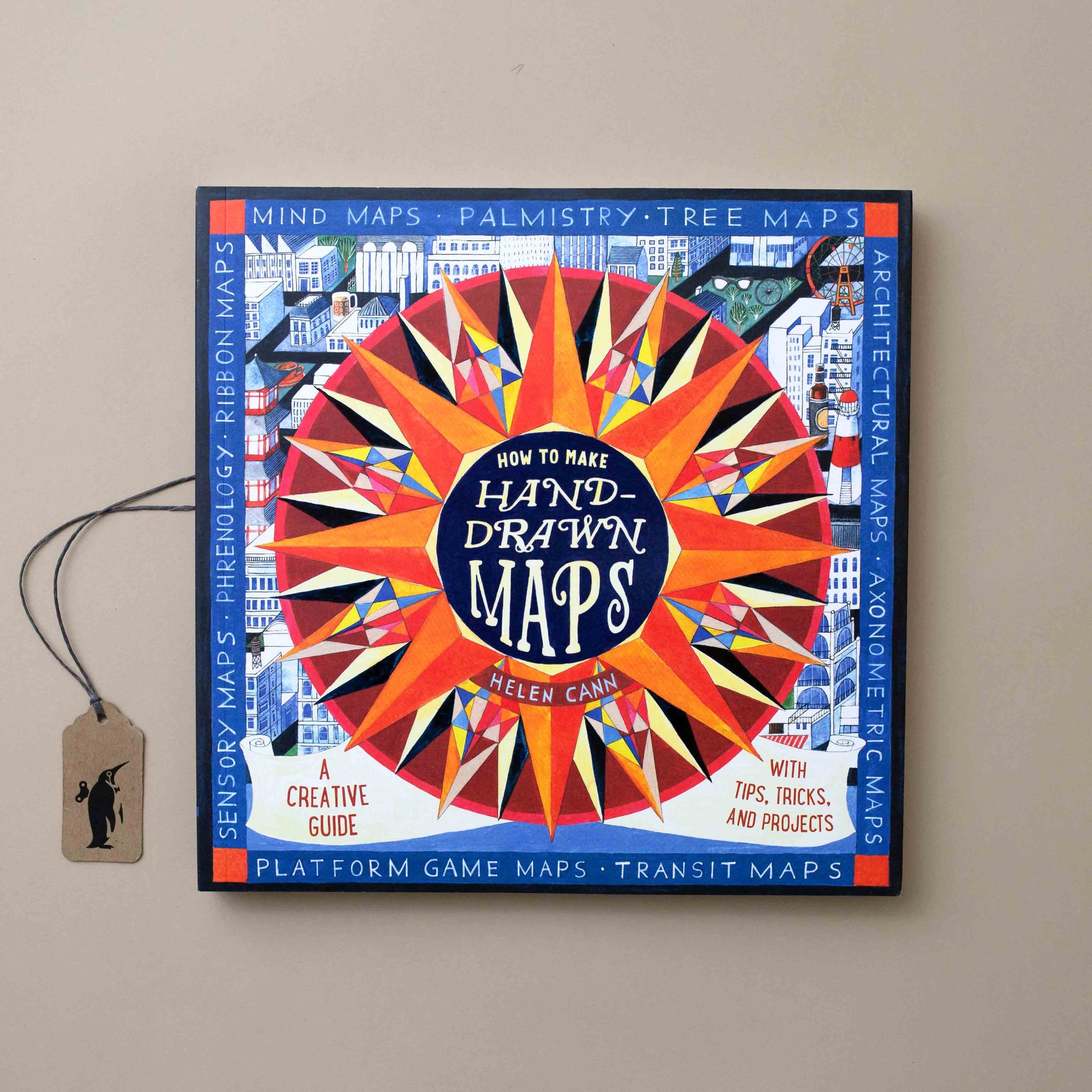The image depicts the cover of a book hung on a gray wall. The square artwork is adorned with a black frame, featuring a blue border along the edge. At the top, the words "Mines Map" are prominently displayed. The central focus of the cover is a large, colorful sun logo, surrounded by numerous orange and red triangles. The text in the center reads, "How to Make Hand-Drawn Maps." The background of the illustration showcases tall buildings, adding an urban feel to the design. Scattered text around the cover includes phrases like "mind maps," "palmistry," "tree maps," "sensory maps," "platform game maps," and "transit maps," all in white letters. On the left-hand side, it states, "a creative guide" in red text, and on the right, it mentions, "with tips, tricks, and projects." Additionally, the book is credited to Helen Kan and includes a notable penguin tag on the left.